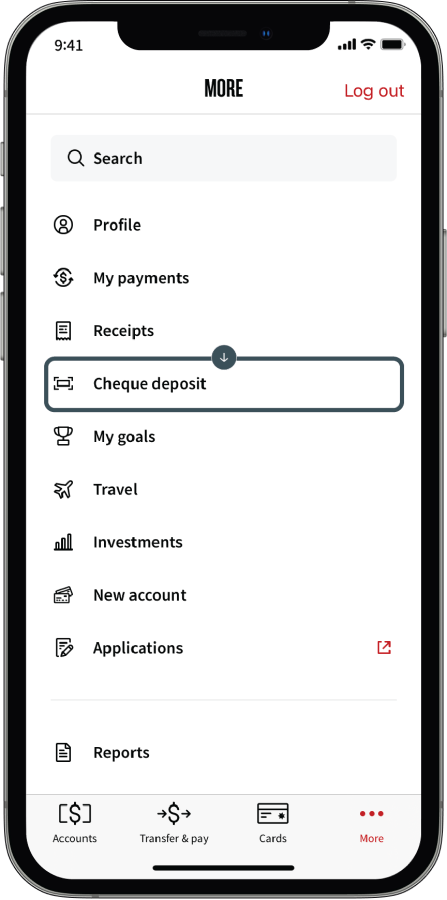**Detailed Caption:**

This is a detailed screenshot from a smartphone showing a banking application interface. At the top, the time displayed is 9:41 AM, accompanied by four bars of cellular service, a Wi-Fi connection icon, and a fully charged battery indicator. The header of the application reads "More," with an option on the right-hand side to log out, marked in red.

Directly below the header is a search bar, followed by a list of user options. The first option listed is "Profile," followed by "My Payments." The third option is "Receipts," succeeded by "Check Deposit," which is highlighted in the interface. Subsequent options listed are "My Goals," "Travel," "Investments," "New Account," and "Applications." Notably, beside "Applications," there is a red box with an arrow pointing to the right.

Below these options is a separate rectangular section labeled "Reports." 

At the bottom of the screen is a light gray footer with several navigation options. From left to right, they include "Accounts," represented by a dollar sign, "Transfer and Pay," illustrated with a dollar sign accompanied by arrows, "Cards," indicated by a credit card icon, and "More," denoted by three red dots on the far right.